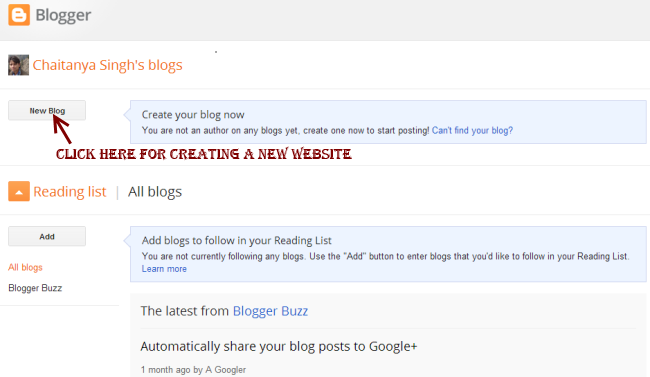This is a detailed screenshot from Blogger, showcasing a blog managed by Chaitanya Singh. Her blog title, "Chaitanya Singh's Blogs," is prominently displayed in orange. An avatar of herself accompanies the title. Below the title, there is an actionable "New Blog" button highlighted by a red arrow with the label, "Click here for creating a new website." Adjacent to the button, a long blue speech bubble encourages users to "Create your blog now." A notification states, "You are not an author of any blogs yet. Create one now to start posting."

Further down in the interface, a blue text link reads, "Can't find your blog?" indicating additional help. The next section titled, "Reading List," in orange, offers options to manage blog subscriptions. An "Add" button is positioned on the left side accompanied by another long blue speech bubble that says, "Add blogs to follow in your reading list." Users are prompted, "You are not currently following any blogs. Use the add button to enter blogs that you'd like to follow in your reading list."

Additionally, a gray box at the bottom, marked "The Latest from Blogger Buzz," highlights updates. This particular entry talks about "Automatically share your blog posts to Google Plus," posted one month ago by a Google user.